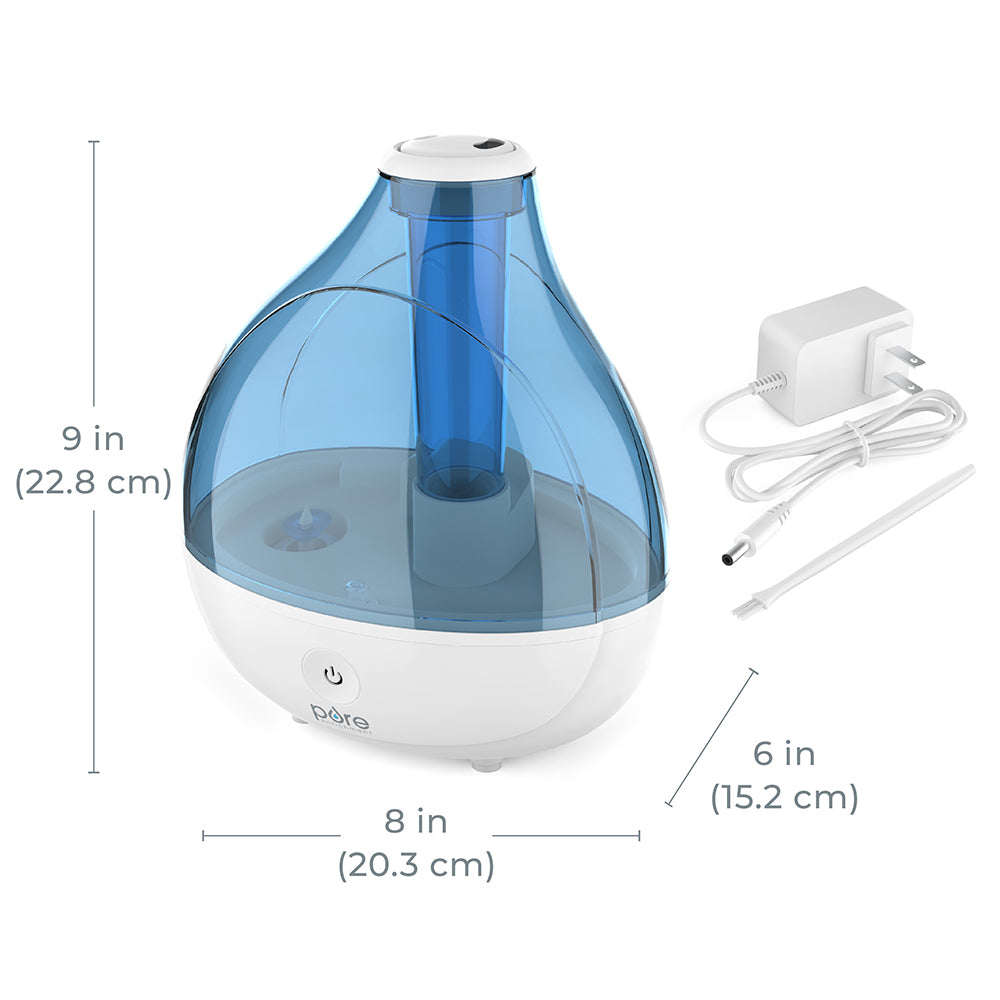This image features an advertising photograph of a compact, tabletop water purifier or humidifier branded as PURE, with the 'U' stylized to resemble a raindrop. The device is placed against a white background, making it appear almost like clip art. The appliance stands at 9 inches tall, 8 inches wide, and 6 inches deep, with a shape reminiscent of a vase or a squished raindrop, where the base is comparatively wider than its depth.

The device itself has a sleek design with a white base that includes an on button, and a top half made of partially transparent light blue plastic. Inside the top half, there is a central blue plastic cylinder that seems to be removable, possibly for maintenance purposes. The product package also includes an American-style plug with a white cord, which is shown coiled and secured with a white band. An additional photo within the image highlights this plug. Moreover, the set comes with a small cleaning brush that looks like a tiny paintbrush, ensuring the device's maintenance is hassle-free.